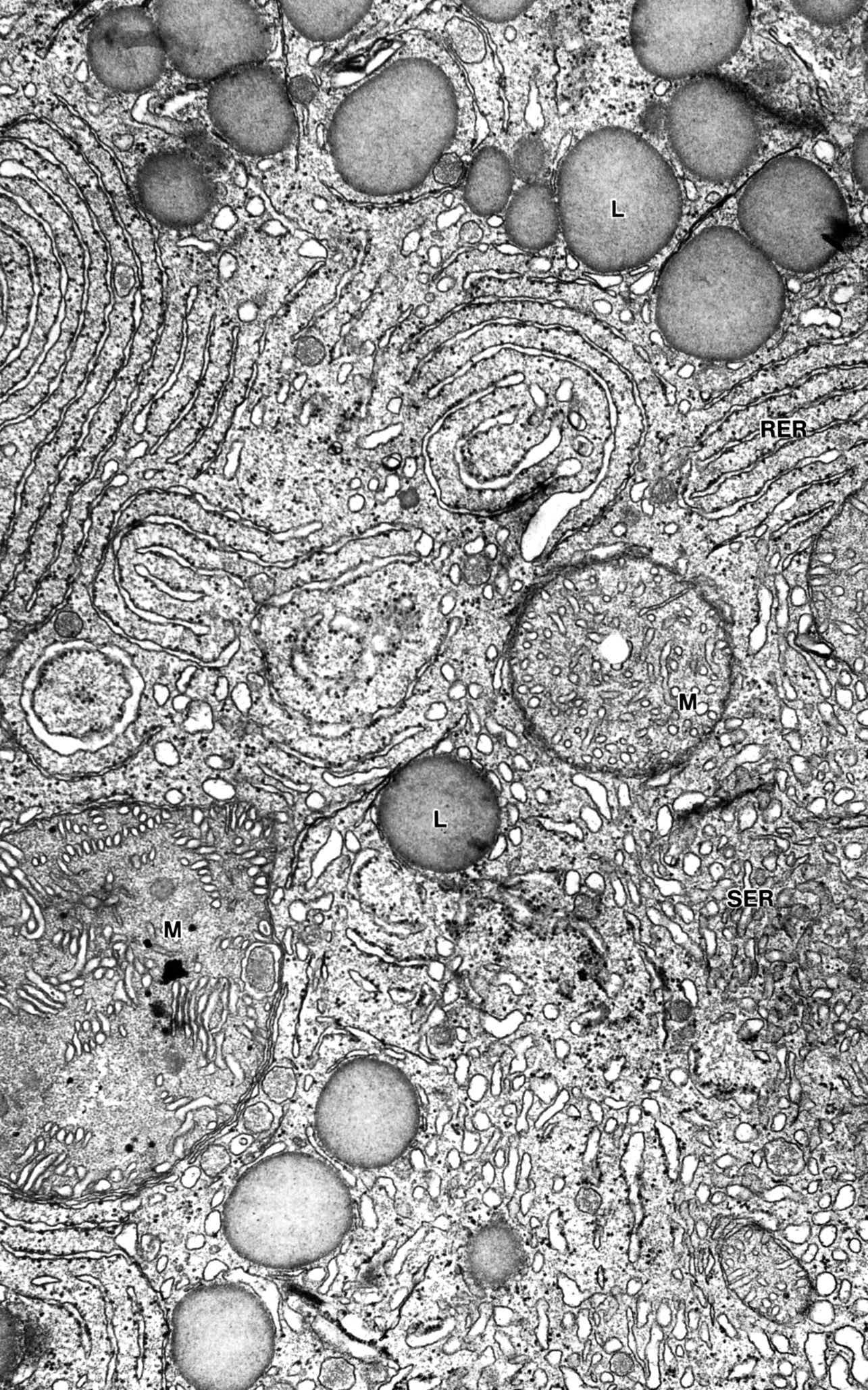This black-and-white image appears to be a highly detailed close-up, potentially captured through a microscope or an electron microscope, though it might also be an art print mimicking such imaging. The composition features a multitude of abstract forms reminiscent of cells or bubbles, primarily circular with white interiors and dark gray to black rims. 

Scattered across the upper part of the image are several of these circular shapes, while a distinctive row runs about a third of the way down from the left to the right. Central to the composition is another prominent circular form. The circles vary in size, some containing plain white interiors, while others house intricate, smaller formations and granular textures. Among these circles, certain ones are labeled with black letters: an "L" is prominent in a circle toward the top right, and another "L" appears in a dark gray circle in the middle. Nearby, a larger circle hosts an "M," with three smaller circles positioned beneath it in a vertical arrangement.

The background, a gradient of gray, is adorned with complex, swirling groove patterns reminiscent of fingerprints. These patterns vary from simple ball-like shapes to elaborate spirals, with major formations in the upper left, central, and right sections of the image. Notably, a dark gray shape resembling a lemon outline is seen in the bottom left, and nearby, another dark gray circle contains an "L" label.

Lastly, towards the right side of the image, the letters “S-E-R” and “R-E-R” can be observed, adding to the array of textual elements present within the circular and oval forms.